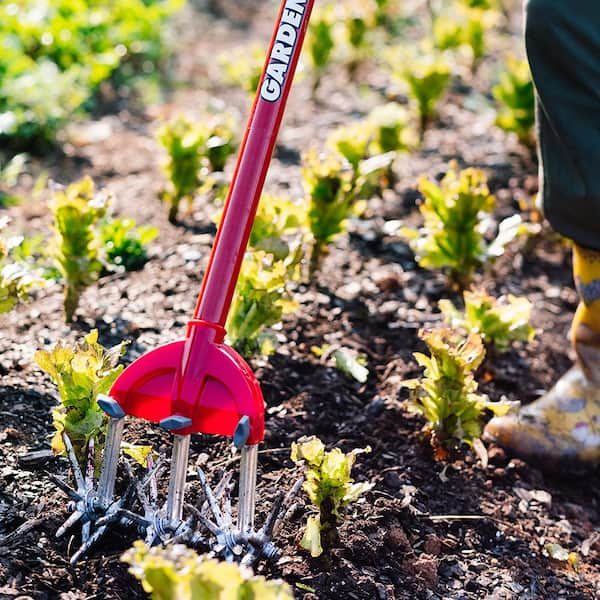In this detailed photograph taken on a sunny day, a person is using a red manual tiller to aerate the soil in a well-maintained garden. The tiller's handle, clearly embossed with the word "GARDEN" in white letters, extends down to wheels equipped with rotary spikes for efficiently cultivating the earth. Only the right booted foot and one leg of the gardener are visible on the far right side of the image. The individual is maneuvering the tool between neatly planted rows of green plants, suggesting they are weeding or preparing the soil. The bright sunlight casts distinct shadows, adding a warm, vibrant ambiance to the scene.